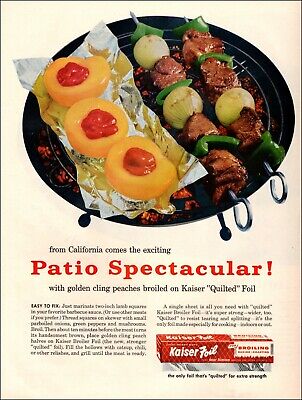The image portrays a vintage magazine advertisement, likely from the 1960s, showcasing a "Patio Spectacular" barbecue theme. The central focus is on a grill featuring two metal skewers with a repeating pattern of green bell peppers, onions, and beef pieces, alongside a foil-covered section holding golden cling peaches slathered in a red sauce. Below the grill image is bold, large red text reading "Patio Spectacular." Accompanying the main visual is a detailed description promoting "golden cling peaches broiled on Kaiser quilted foil," emphasizing the appeal of using Kaiser foil for grilling. At the bottom of the ad, there's an image of a red box of Kaiser aluminum foil, reinforcing the product being advertised.